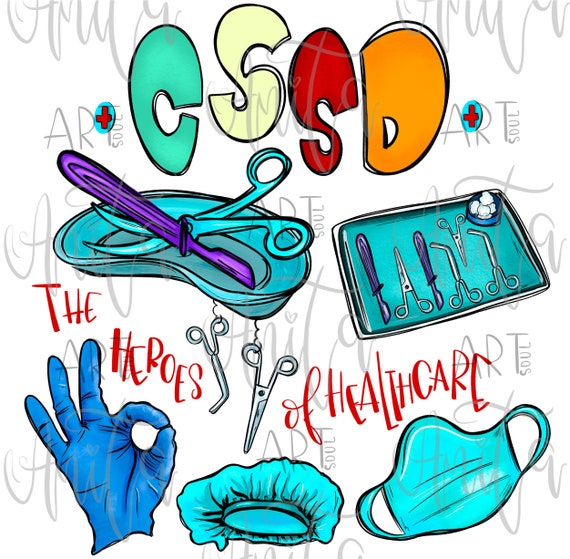This vibrant, surreal illustration features a variety of colorful surgical tools and equipment set against a white background adorned with faint gray lettering. At the top, the letters "CSSD" are displayed in a whimsical, distorted font with each letter in a different hue: turquoise, light green, red, and orange. Flanking the text are hospital plus signs inside turquoise circles. 

Below this heading, a blue kidney-shaped tray holds a matching pair of teal scissors and a purple scalpel. To the right, another tray contains four silver hemostats, additional purple scalpels, and a few cotton balls. Beneath these central images, the phrase "The Heroes of Health Care" is prominently written in bold red text. 

Directly under this, three items are illustrated: a blue gloved hand making an OK symbol, a light blue surgical cap, and a matching light blue surgical mask. Scattered throughout the image is a watermark reading "Anita and Art Sol." The piece is detailed with an array of vivid colors and is rendered in a playful, exaggerated style that blends the seriousness of its surgical theme with a cartoonish aesthetic.